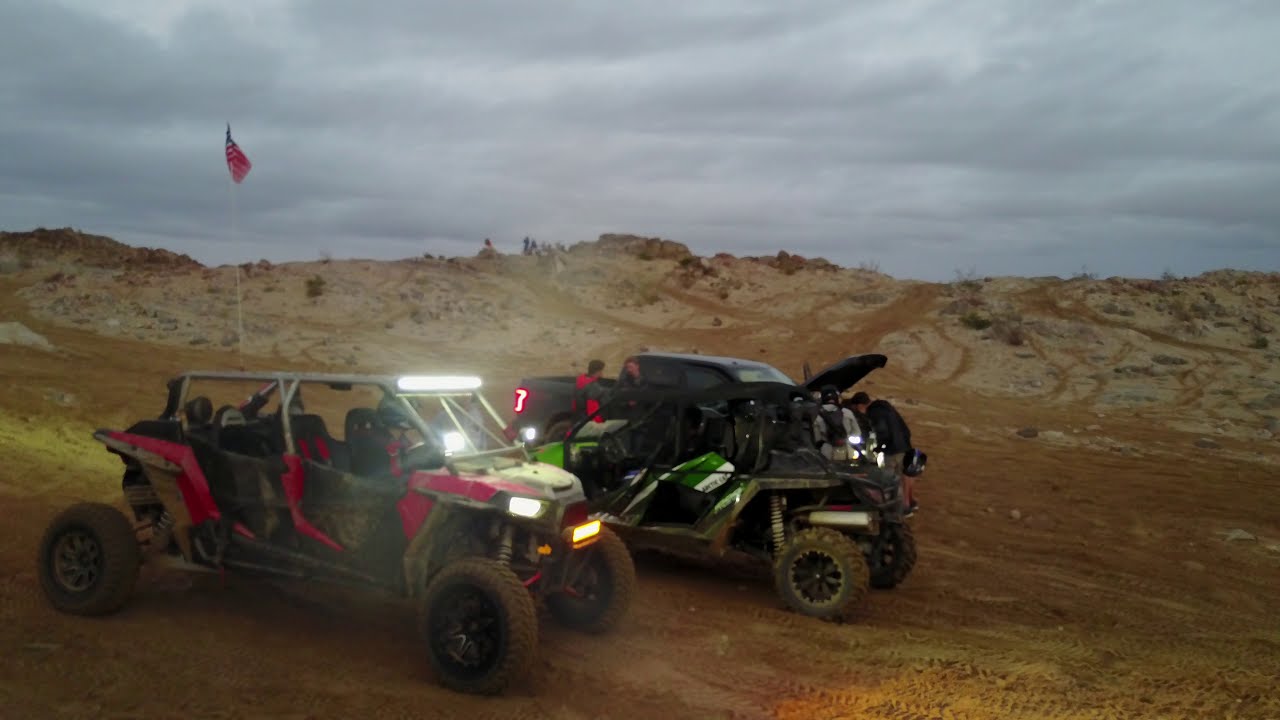The rectangular photograph captures a rugged desert scene dominated by soft sand and clay dirt, punctuated by a few scraggly plants. In the foreground, two large all-terrain vehicles (ATVs) draw immediate attention. The front ATV, red and gray with a light bar illuminated, is a four-seater and positioned on the left side, facing right. Behind it to the right, a black ATV with green and white stripes, also presumably a four-seater, faces left. Further back, a black pickup truck, taillights glowing red, stands with its hood popped. Around the truck, four men are engaged—two by the open hood and two conversing at the rear door. Above the scene, a tall white flagpole hoists an American flag fluttering gently. The background reveals expansive sand dunes, where a few indistinct figures are visible at the crest. The sky, thick with gray and white clouds, suggests impending rain, casting a dim, evening-like light over the entire landscape, with vehicle headlights sharply piercing the growing twilight.